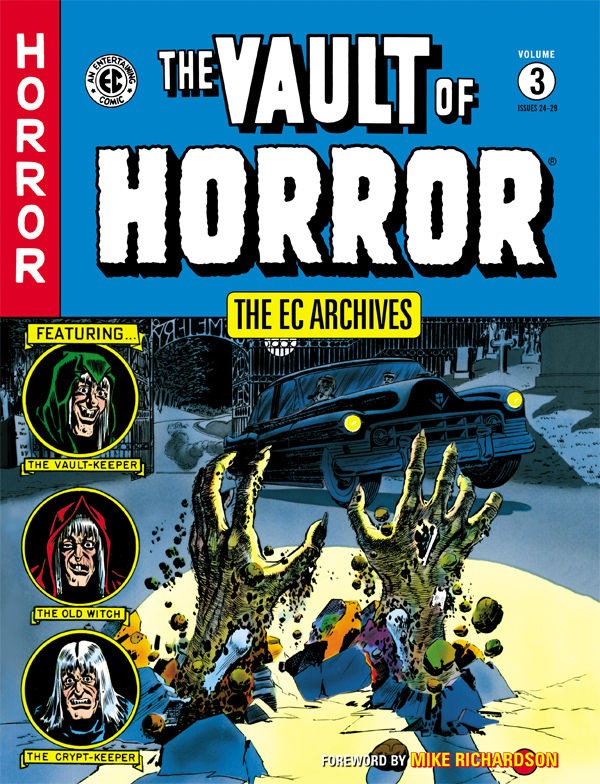The cover of this comic book, clearly titled "The Vault of Horror," is vivid and rich in detail. On a small vertical red banner along the top left, the word "Horror" is prominently displayed in white letters. Directly below, on a blue background, it reads "The Vault of Horror" in a bold, comic book-style font, with "Volume 3" marked in corresponding white text and numerals. The yellow banner beneath this segment proudly announces "The EC Archives." 

The cover also features an "Entertainment Comic" stamp and includes a prominent byline stating "Foreword by Mark Richardson" at the bottom right. Along the left side, three distinct characters are highlighted: the Vault Keeper, the Old Witch, and the Crypt Keeper. The Vault Keeper, depicted as an older man with a half-insane look and wearing a green hood, is followed by an image of the Old Witch, who appears more like a man with white hair under a red hood. Lastly, the Crypt Keeper sports a blue cape and white hair, without a hood.

Dominating the central imagery of the cover, two green hands emerge menacingly from the ground in a graveyard setting, complete with a fence and headstones in the background. A 1930s-style dark sedan is depicted hurriedly driving past these eerie hands, accentuating the horror theme. The combined visual elements and vibrant colors create a captivating and chilling introduction to this volume of horror tales.